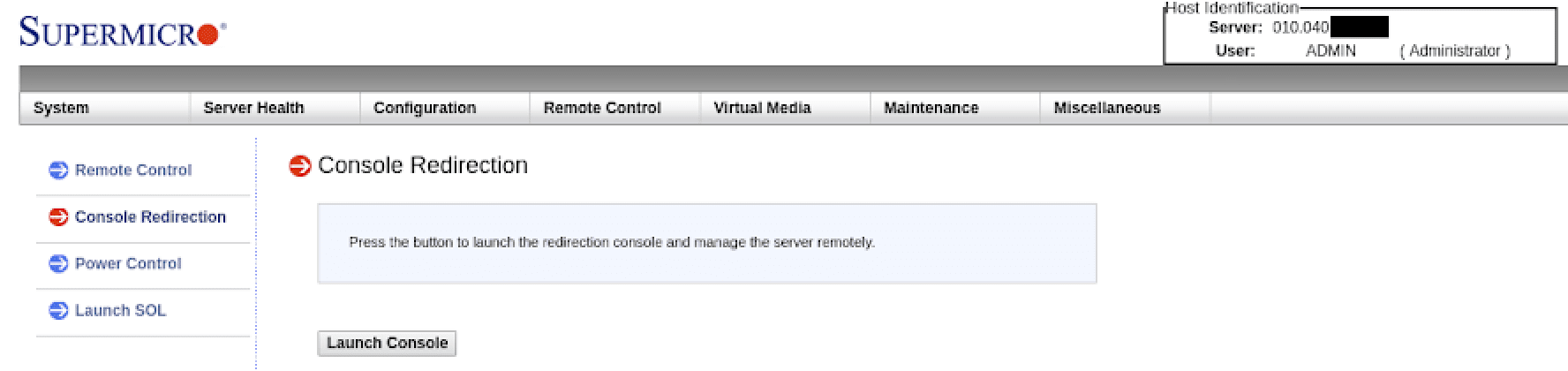This screenshot is from a website interface for managing servers. In the top left corner, the brand name "Super Micro" is displayed, with the "O" in "Micro" represented as a red dot. In the top right corner, it reads "Host Identification, Server 010.040," with a section that has been blacked out for confidentiality. Beneath that, it lists the user as "admin administrator."

A horizontal menu bar stretches across the screen, offering various options: System, Server Health, Configuration, Remote Control, Virtual Media, Maintenance, and Miscellaneous. Along the left side of the interface is a vertical menu. The options include Remote Control, Console Redirection (which is currently selected), Power Control, and Launch SOL.

To the right of the vertical menu, there is a red circle with a white arrow pointing to the right next to the text "Console Redirection." Below this, there is a long gray rectangle instructing users to "press the button to launch the redirection console and manage the server remotely." Under this instruction, another gray rectangle includes the words "Launch Console" in black letters.

The screenshot is purely of a graphical user interface with no photographic elements, people, animals, birds, plants, flowers, or trees present.